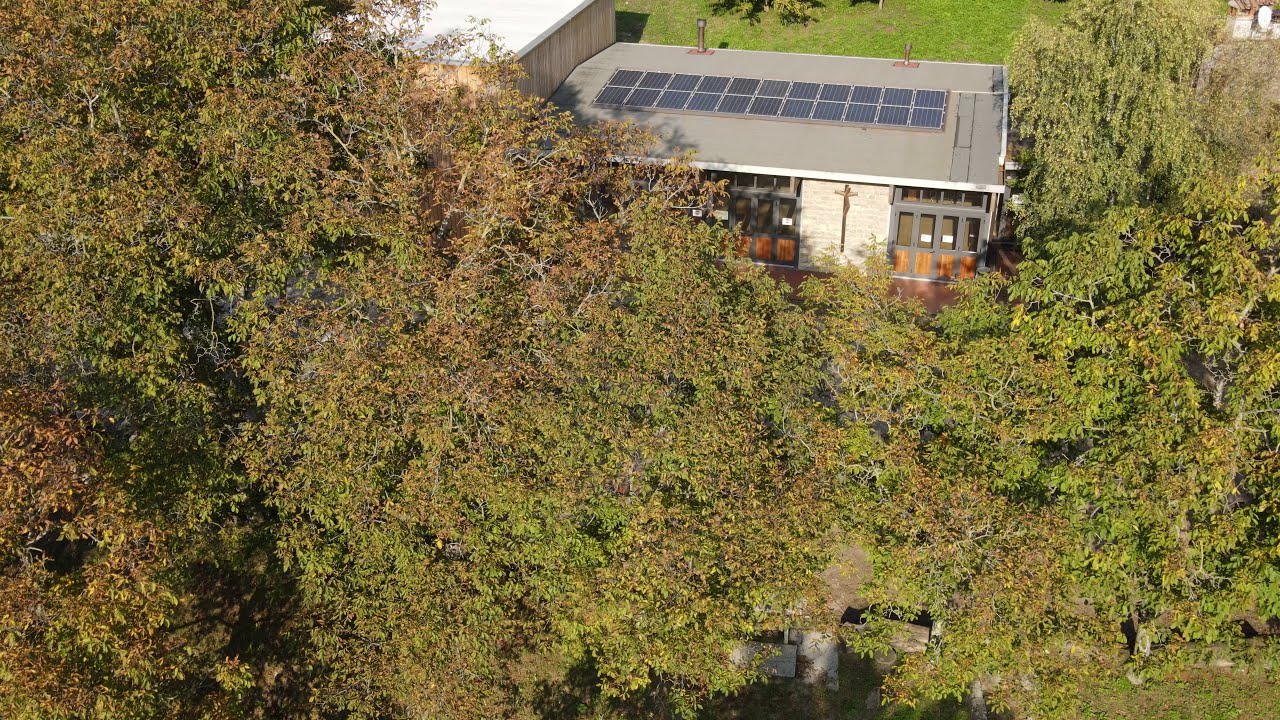An aerial photo captures a landscape featuring a large building, partially obscured by dense, late-summer or early-fall green and brown foliage. The building, potentially a church due to the prominent brown cross on its white brick facade, has a gray, flat roof adorned with black solar panels. Adjacent to this structure is a smaller, plainer building with a white roof, which is partially hidden by the tree canopy. The sunny, midday light casts minimal shadows across the scene.